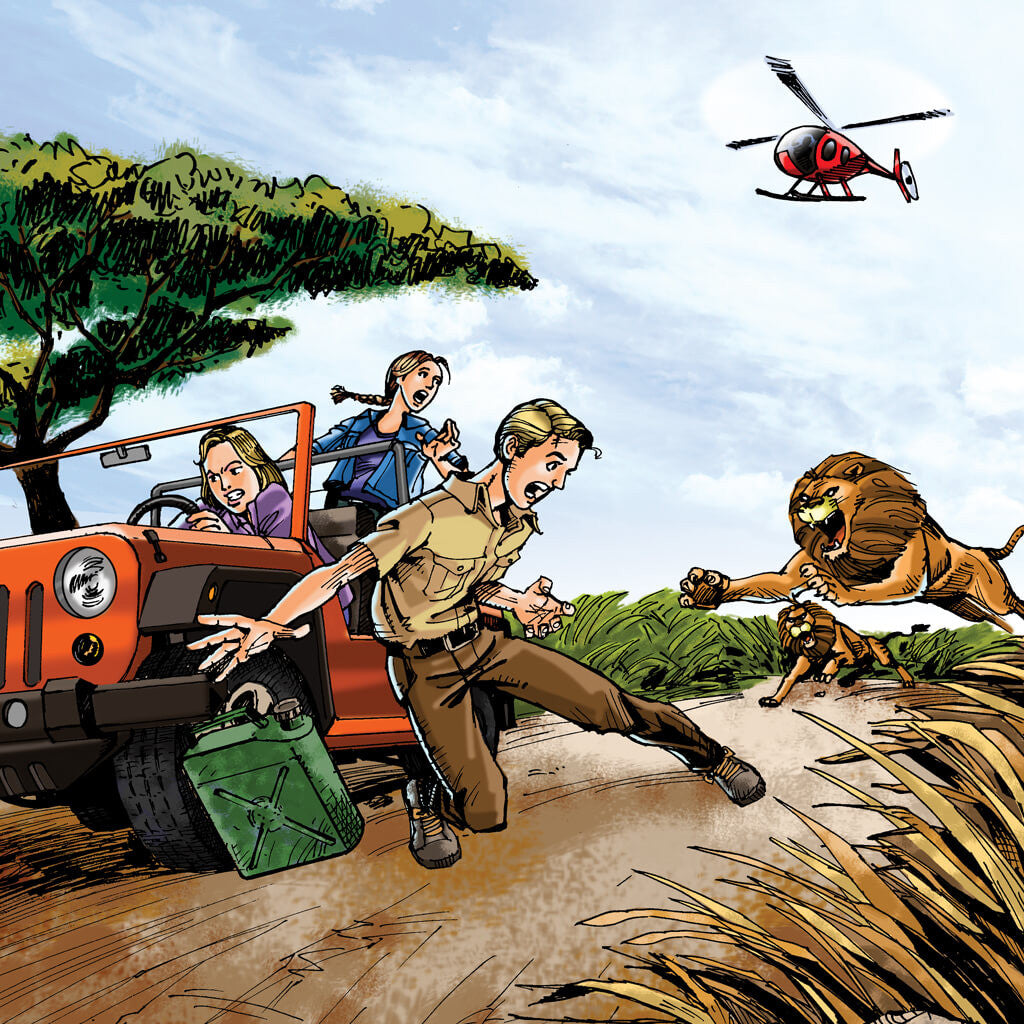This vibrant cartoon drawing depicts a tense safari scene on a dirt road. In the right-hand corner, a black and red helicopter soars through a blue sky adorned with a mix of gray and white puffy clouds. On the left side of the image stands a green, somewhat flat tree next to a red Jeep. Behind the wheel of the Jeep is a woman, while a man in a brown shirt and pants is just outside of the vehicle. He is in the process of dropping a green gas can, likely intended to refuel the Jeep, but his attention has been abruptly diverted. He is falling to one knee in alarm as two ferocious male lions emerge from the grasses alongside the road, mouths open wide and claws extended. One lion is caught mid-leap, aiming directly at the man, while the other follows closely behind on the ground. A girl with blonde hair styled in a long braid, wearing a blue jacket and pink shirt, stands in the back of the Jeep, yelling in terror. The setting is completed by stretches of green grasses on the left and yellow-orange stalks on the right, enhancing the wild and perilous atmosphere of this safari adventure.